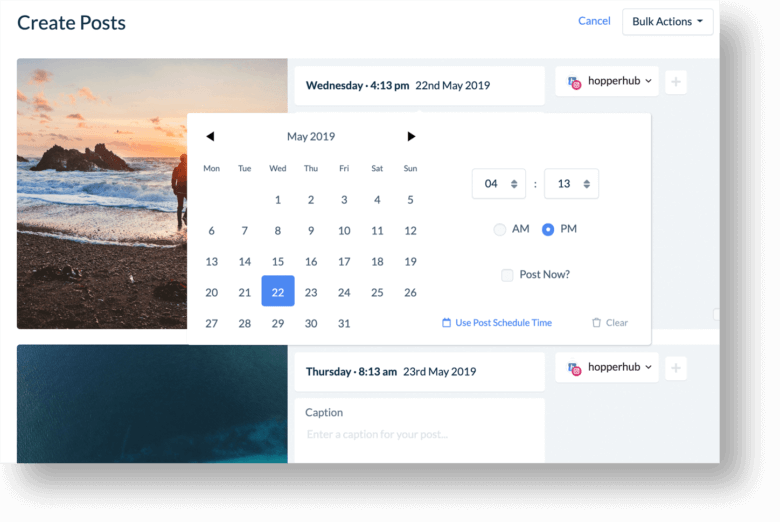The image is a detailed screenshot of a post scheduling interface, likely for a social media or blog platform, centered around a tool called Hopper Hub. The interface is divided into three distinct sections:

**Left Section:**
- Features a partially visible stock photo of an individual on a beach. 
- Below this image is another box with a green border at the page's bottom.

**Middle Section:**
- Begins with a date search box revealing "Wednesday, 4.13 PM, 22nd May, 2019."
- A larger, superimposed calendar box displays the same date, featuring navigation buttons to browse through the calendar and a time selector where "04.13 PM" is already entered. 
- Below the time selector, it shows "Thursday, 8.13 PM, 23rd May, 2019," with a field designated for adding a caption.

**Right Section:**
- This column is the simplest, branded with "Hopper Hub" at both the top and bottom.
- Includes options for bulk actions and a cancel button adjacent to the "Create Post" header.

Overall, this screenshot provides a comprehensive view of the scheduling functionalities in the Hopper Hub interface, demonstrating how users can organize and time their posts.